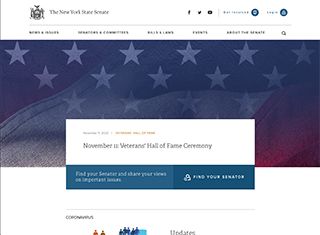Detailed Caption:

This screenshot captures a website page featuring a prominent headline at the top reading "The New York". Central to the image is a flag adorned with horizontal blue, white, and red stripes. The flag also features an arrangement of stars set in distinct rows: two stars in the first row, followed by three stars in each of the next three rows, and concluding with two stars in the final row. Below the flag, the text announces an upcoming event: "November Veterans Hall of Fame Ceremony". Towards the bottom of the screenshot, there is a 'Find' button, alongside an 'Updates' section. Additionally, a logo depicting a group of people is visible, symbolizing community or organizational affiliation. The text in the image appears blurry and difficult to read clearly.